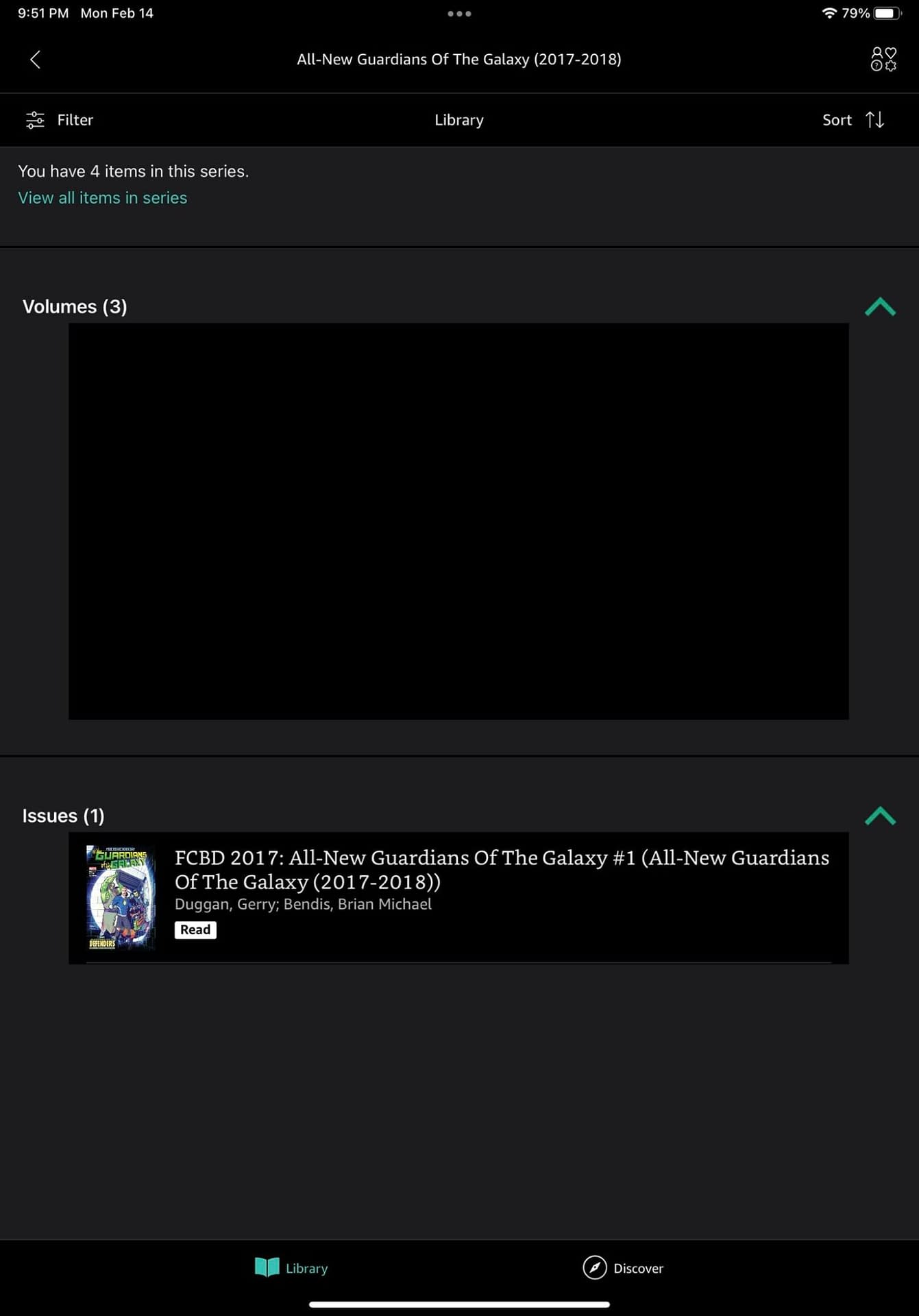The image features a detailed black rectangular interface with various white and colored text elements arranged vertically. At the top center, there are three horizontally aligned white-gray dots. Just below these dots, the text "All-New Guardians of the Galaxy (2017-2018)" is displayed prominently. Below this, the word "Library" is centered, with "Filter" positioned to its left. On the right side of "Library," there is the word "Sort," accompanied by two arrows indicating up and down directions.

The next line reads, "You have four items in this series," positioned directly below "Filter." Beneath this text, a light blue link states, "View all items in series." Further down on the left side, the text "Volumes (3)" is displayed. The remaining large section of the box appears empty and black, providing a stark contrast to the text above.